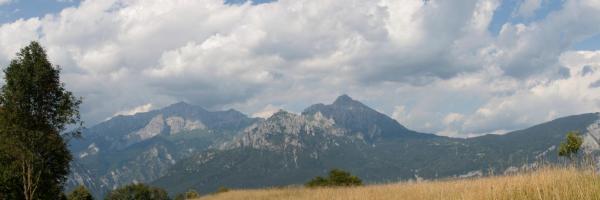This photograph captures a picturesque outdoor natural setting featuring a vast, flat grassland in the foreground, filled with tall, beige, dry wheat-like grass. Scattered throughout this ground area are a few deep green trees and bushes. Beyond this grassy plain lies a distant mountain range, with some peaks topped with snow, transitioning to bare stone grey hues further down. Above the mountains, a dramatic sky is predominantly covered with large white and grey clouds, with only glimpses of blue sky peeking through. The photo, a rectangular frame with a longer width than height, showcases the mountains desaturated from the ground due to atmospheric pressure, rendering a serene yet majestic panorama.